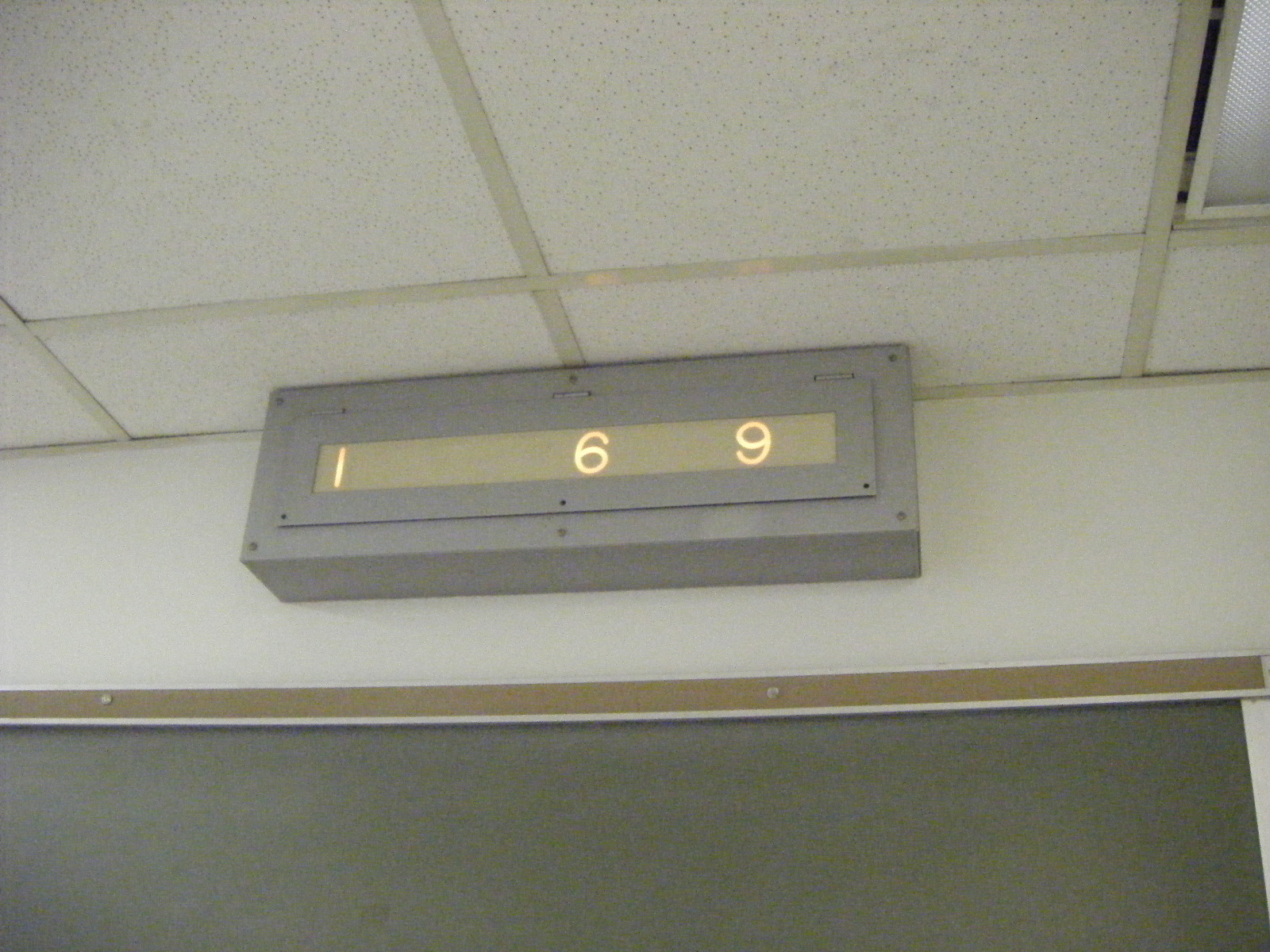The photograph depicts the upper section of an interior wall, possibly in a classroom or similar setting, with white ceiling panels that have black specks, framed in a yellowish or tannish white color. A light fixture is visible on the right side, with a noticeable gap showing a black area between the panel and the light. On the white wall below the ceiling, there is a gray-colored metal box, securely screwed in place, displaying illuminated numbers: a "1" on the left, a "6" in the center, and a "9" on the right. This arrangement suggests it is an indicator panel for an elevator. Below this panel, a large door frame area is visible, featuring brown trim secured with silver screws, and a dark gray door, which is likely the elevator door.